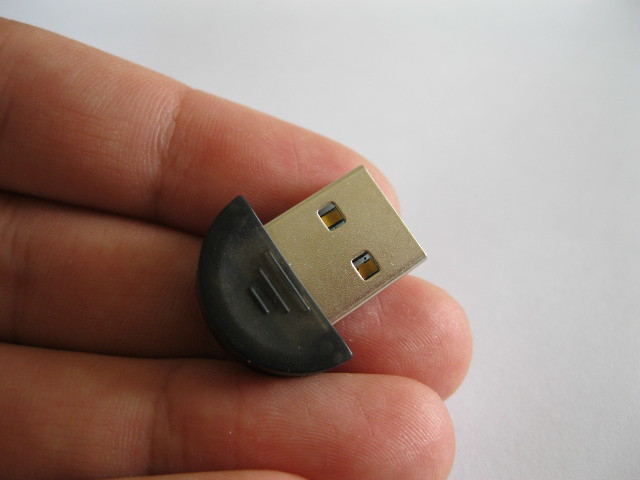A close-up image features a left hand extending from the left side of the frame, with the index, middle, and ring fingers holding a Bluetooth USB stick. The background appears to be a white or off-white surface, casting a slight shadow that gives it a partially gray hue. The USB stick is distinctly identifiable by its black semi-circle base adorned with three line patterns, providing a grip. Above the base, a silver metallic section with two square cutouts reveals internal white lines and a central yellow detail, making it potentially a receiver for a wireless device. The image is detailed enough to capture the textures of the fingers, including the grooves of the fingerprints and the bending lines at the knuckles.